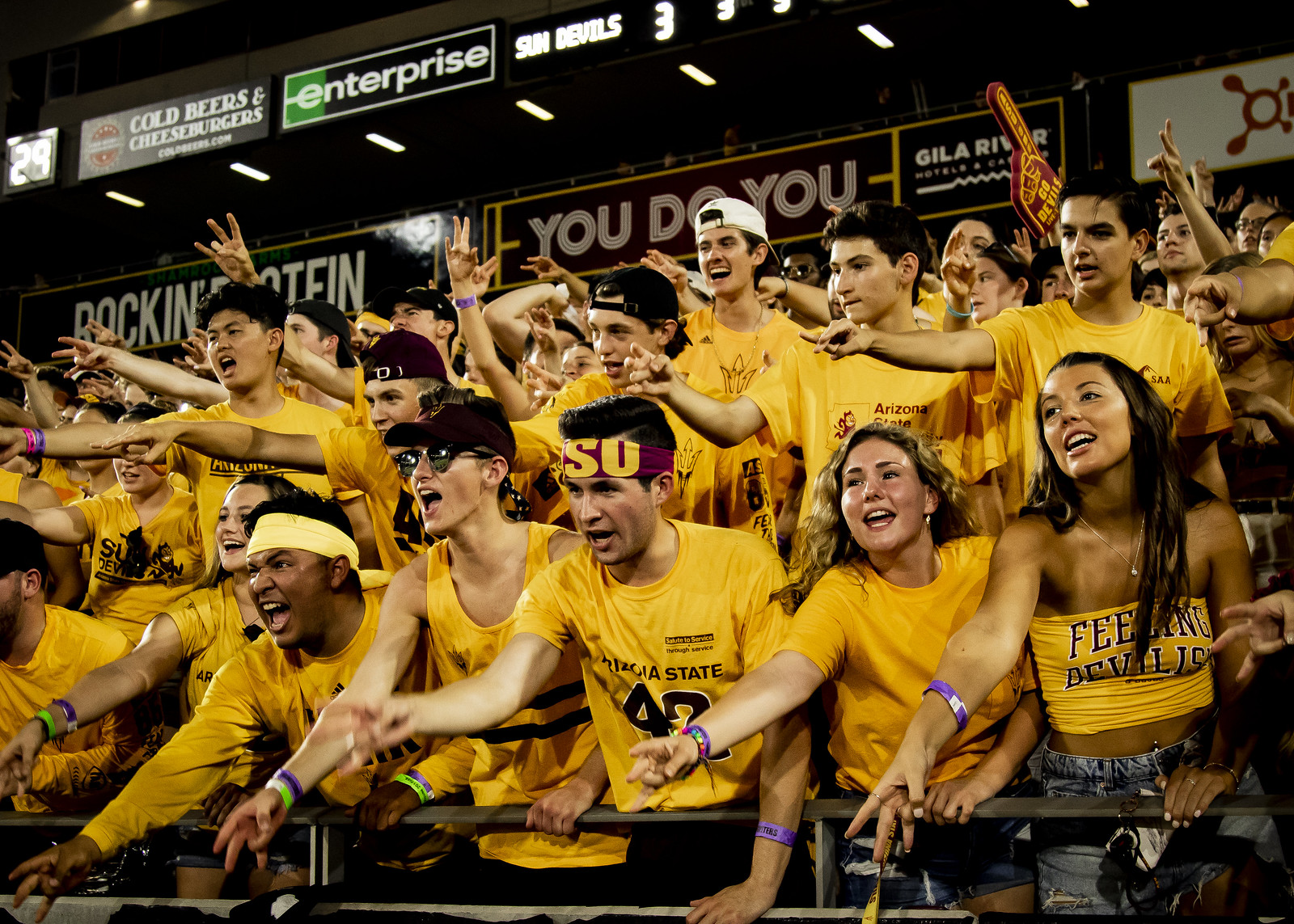The photograph captures a close-up section of an enthusiastic crowd at an Arizona State University game. The scene is dominated by college-age students, most likely in their early 20s, all donned in yellow t-shirts or muscle shirts, some of which bear "Sun Devils" insignia. The crowd is packed into the bleachers of an arena, with many fans standing and visibly engaged in the event. Many of the students sport backward baseball caps, and some wear sunglasses or purple and green paper wristbands. In unison, they stretch their right hands forward, forming a scissor-like gesture with their fingers, all focused intently on the action happening off to the left. The background of the image features advertising signs for cold beers, cheeseburgers, Enterprise Rent-A-Car, and Gila River Hotels, adding to the vibrant atmosphere of the game.